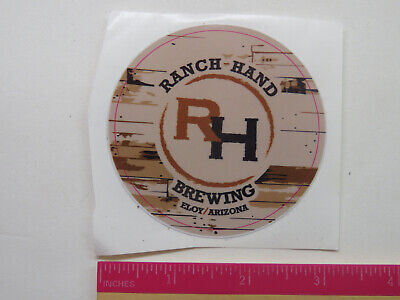The image depicts a round sticker fixed to a slightly creased white mat. The mat is measured with a pink ruler at the bottom, indicating that the sticker is just over three inches in diameter. The sticker features a design resembling weathered, light-colored wood with darker brown stripes, giving it a rustic, wooden appearance. At the top of the sticker, in semicircular black text, is the phrase "Ranch Hand." Below it, in an inverted semicircle, it reads "Brewing, Eloy, Arizona." Centrally positioned is a logo consisting of a brown "R" overlapping a black "H," encased within two brown semicircles.